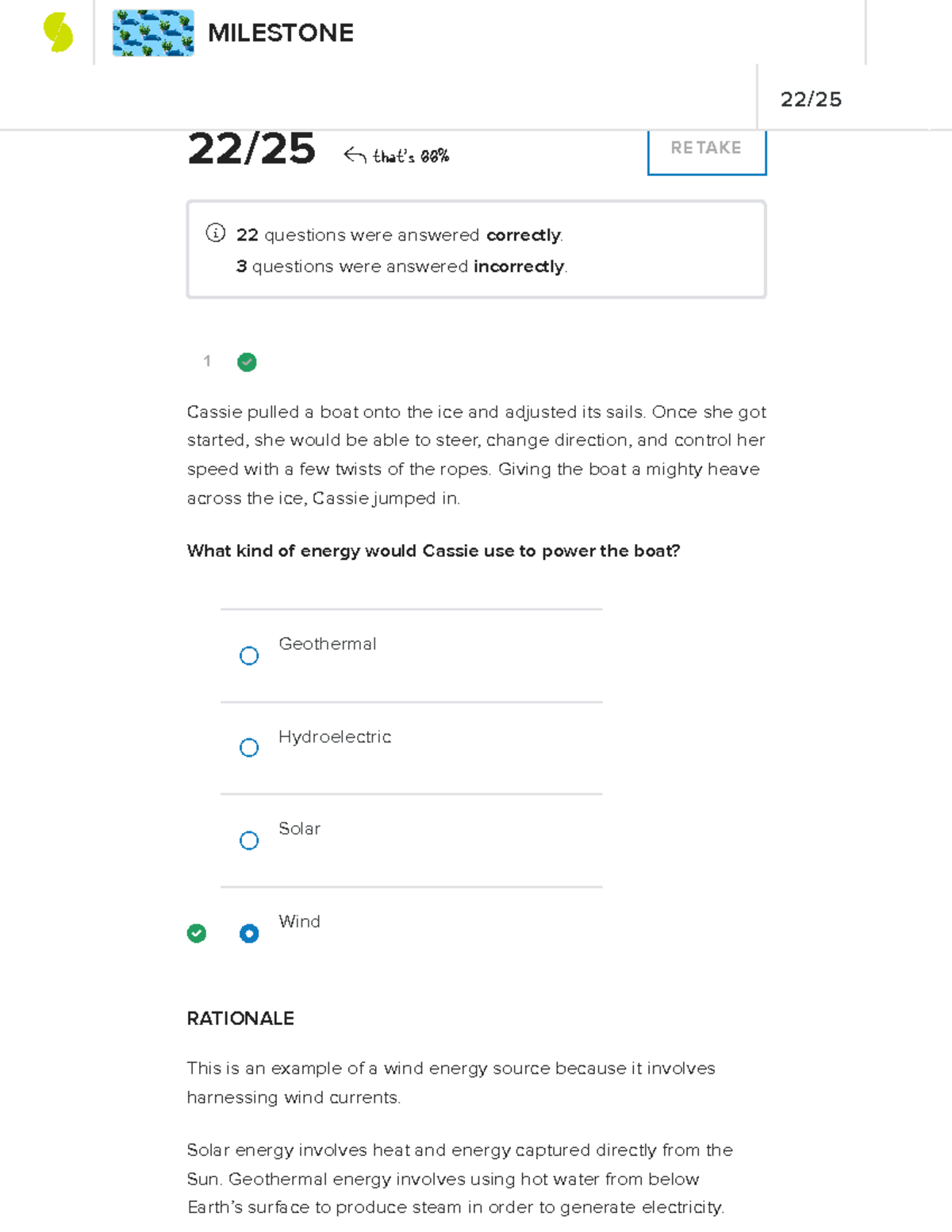This image is a screenshot displaying an online test administered by an entity called Milestone, identifiable by its logo located in the top left corner. The Milestone logo consists of two light green half circles positioned apart, paired with a blue square icon representing potential answers. The test in question is numbered 22 out of 25. The respondent achieved a score of 86%, correctly answering 22 out of 25 questions.

Visible on the screen is an option to retake the test, which is grayed out but still selectable. Below this, there is a summary indicating that 22 questions were answered correctly while 3 were answered incorrectly. The image goes into detail about question number one, which has been answered correctly by the test taker, as indicated by a green check mark.

The question reads: "Cassie pulled a boat onto the ice and adjusted its sails. Once she got started, she would be able to steer, change direction, and control her speed with a few twists of the ropes. Giving the boat a mighty heave across the ice, Cassie jumped in. What kind of energy would Cassie use to power the boat?" 

The response options provided were: 

- Geothermal
- Hydroelectric
- Solar
- Wind

The correct answer, "Wind," is highlighted on the test. Below the question and answer is an explanatory rationale stating, "This is an example of wind energy source because it involves harnessing wind currents. Solar energy involves heat and energy capture directly from the Sun, while geothermal energy involves using hot water from below the Earth's surface to produce steam in order to generate electricity." The rationale does not provide additional commentary on hydroelectric energy.